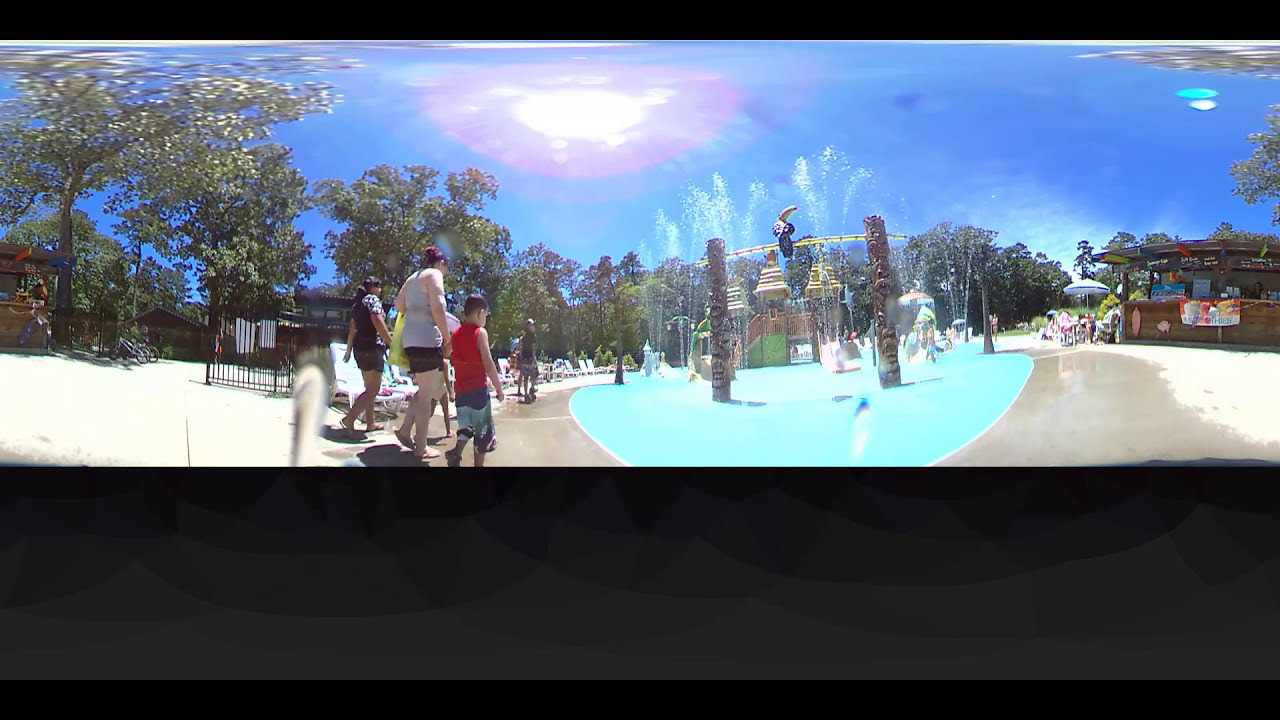The image depicts a sunny, cloudless day at a lively water park, with a clear blue sky and a bright atmosphere. A family is seen walking towards the center of the park, which features an interactive fountain area where water sprays up from the ground, providing a refreshing splash for visitors on a hot day. The family consists of a man, a woman, and a young boy wearing a red t-shirt and shorts, strolling together amidst the playful water jets. The man on the left is dressed in black, while the individual in the middle sports white and black trunks. Behind them, a concession stand nestled among trees offers refreshments, likely including treats like snow cones, indicated by its colorful umbrella. The park is equipped with various structures and poles that appeal especially to children, and the overall arrangement suggests a vibrant and inviting setting for family fun.